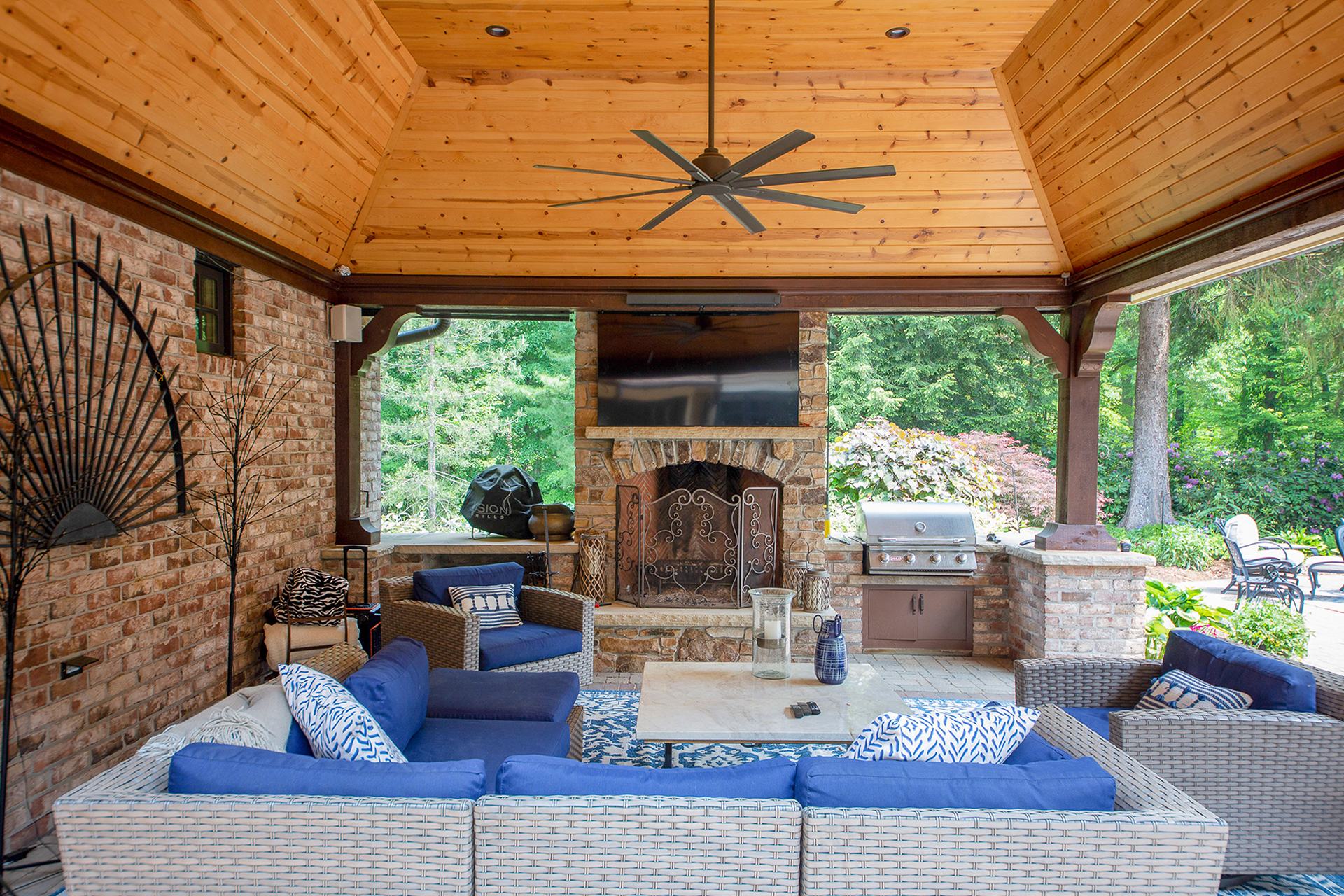This image depicts a meticulously crafted indoor-outdoor patio, showcasing an elegant transition from home to nature. The ceiling, made of rich stained wood, features two recessed lights and a prominent eight-blade ceiling fan suspended by a long shaft. The semi-enclosed space is anchored by an inviting brick fireplace at the center, above which is mounted a TV and sound bar, making it a perfect spot for entertainment. Surrounding it is a half-wall enclosure, except to the right where the patio opens to the outdoor environment, revealing a garden and woodland edge.

The patio boasts an outdoor kitchen with a large stainless steel barbecue grill, encased in sophisticated stonework, hinting at high-end materials used throughout. Complementing this area is an array of wicker-style furniture with a coastal touch: a sofa, two armchairs, and a loveseat, all adorned with plush blue cushions and accented by blue and white throw pillows. A square coffee table with a travertine stone top sits centrally, decorated with a blue vase and a clear white candle holder. A matching decorative rug ties the seating area together with blue and white designs. Further in the background, additional wrought iron patio furniture provides extra seating options. The entire layout offers a seamless expansion of living space, blending comfort and luxury against the backdrop of nature.